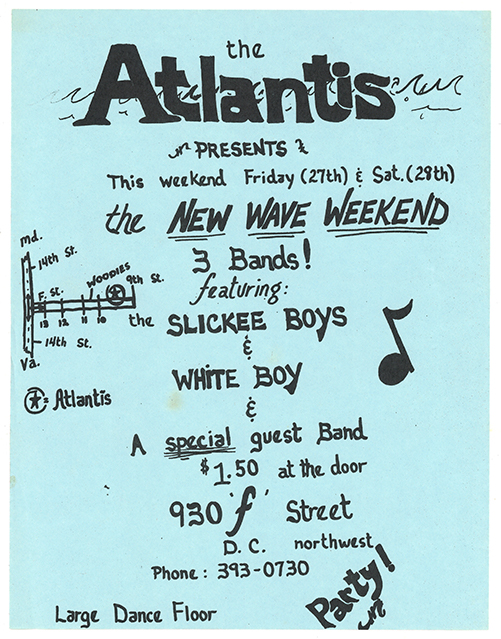This is an invitation or promotional poster for an event called "New Wave Weekend" presented by The Atlantis. The poster features a light blue background with black text. At the top, "The Atlantis" is written in bold. The event is scheduled for Friday, the 27th, and Saturday, the 28th, and will feature three bands: the Slicky Boys, White Boy, and a special guest band. Entrance is $1.50 at the door. The event will be held at 930 F Street, D.C. NW. For inquiries, the contact number is 393-0730. 

The poster highlights that there is a large dance floor available and encourages attendees to "party" in bold letters. On the right side, there is a musical note illustration. On the left side, there is a small map providing directions, showing a vertical line labeled "MD 14th Street" and a horizontal line with notches for "F ST, 13, 12, 11, 10." There is a circle with a star inside, indicating the location. The name "Atlantis" is written on the left, adding a directional guide to the diagram.